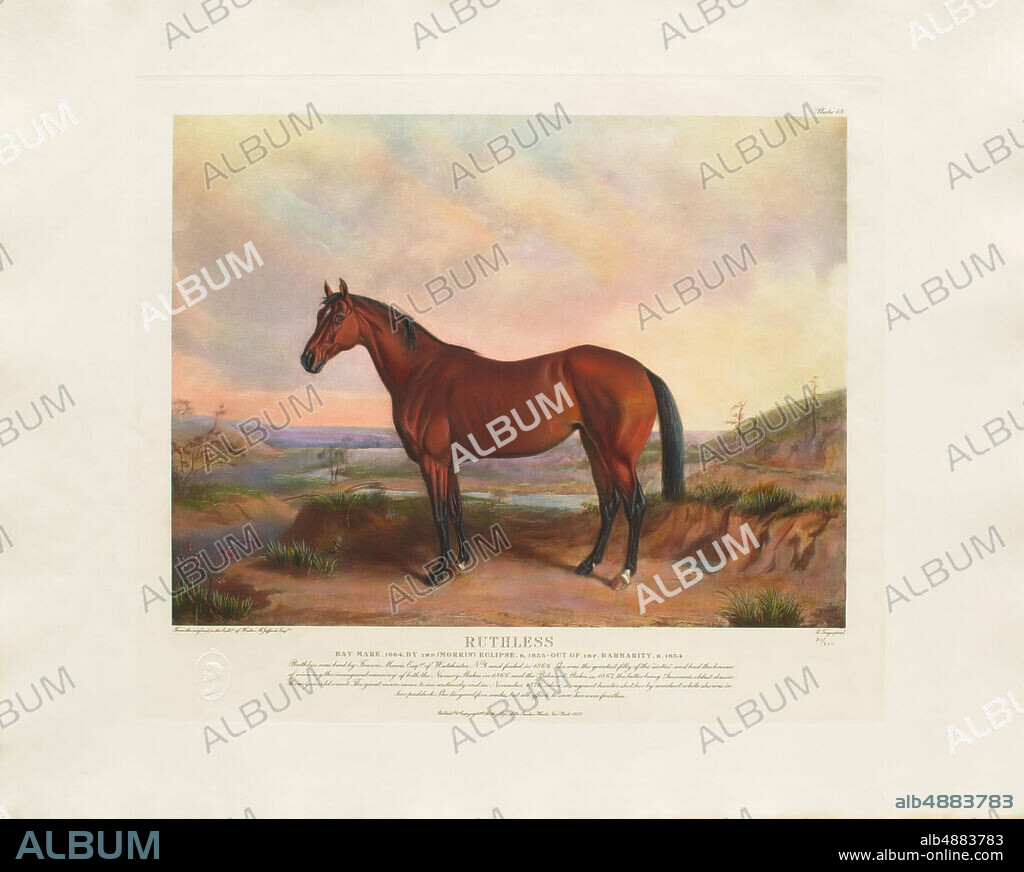This image displays a detailed painting of a dark brown horse, standing on a dirt surface with its head slightly turned towards the camera. The horse features a black mane and tail, with black coloration extending from its knees down to its hooves. It is positioned against a backdrop that includes a serene lake beneath its belly, flanked by patches of greenery, and a sky blending hues of blue, yellow, and red.

The painting is framed with a peach-colored border that extends about an inch inward on all four sides, and a black border at the bottom, approximately a quarter-inch wide. In the bottom right corner of this black border, in blue letters, it reads "ALBUM". Directly beneath is the ID "ALB4883783" along with the website "www.album-online.com".

Additionally, the image is heavily watermarked with the word "ALBUM" repeated multiple times in white and gray across the entire photograph. Below the horse painting, there is some text that reads "RUTHLESS" followed by several lines of smaller, unreadable text. This image is likely a watermarked screenshot or a screen grab, emphasizing its digital reproduction.